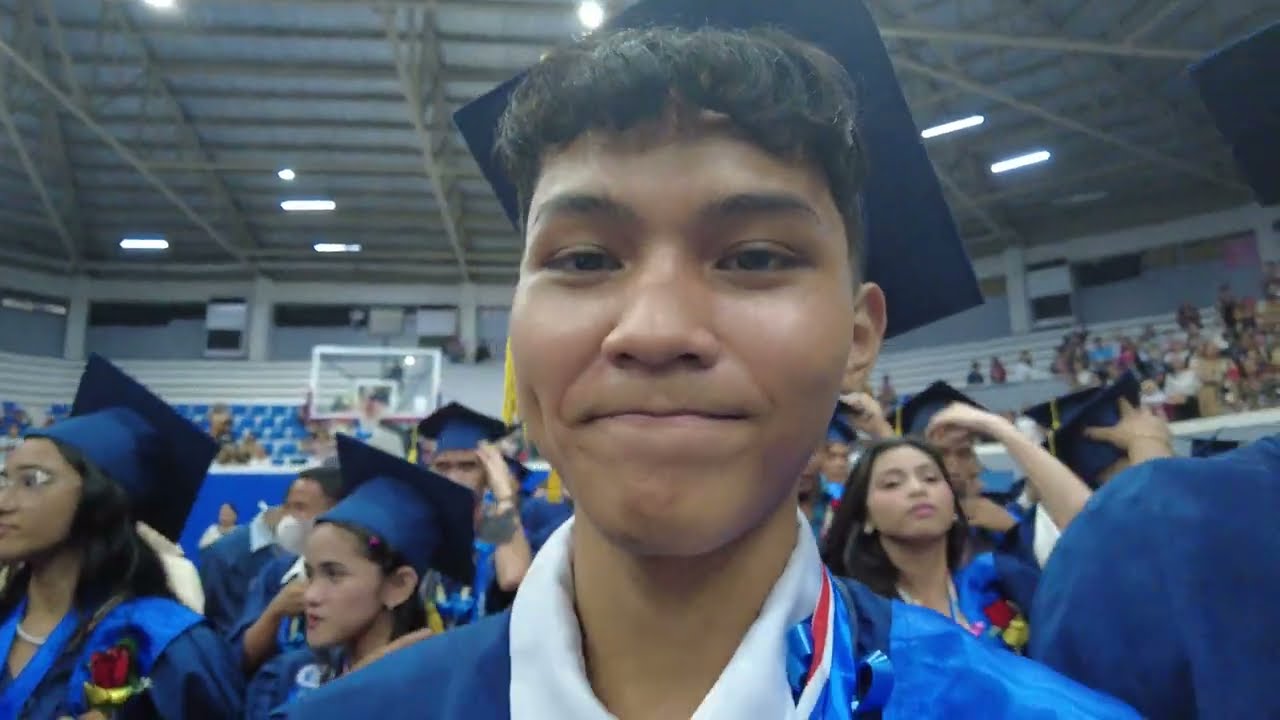A selfie taken during a graduation ceremony in a gymnasium filled with fellow graduates captures a proud moment for a young man. The young man, with curly black bangs, thick black eyebrows, and dark skin, wears a navy blue graduation gown with royal blue trim and a blue graduation cap with a yellow tassel. He confidently smiles with his lips closed, displaying a hint of a dimple on the right side of his face. The background reveals a bustling scene of graduates of various races and genders, all dressed in similar blue caps and gowns. Visible behind them are the gymnasium's features, including a basketball hoop over the young man's right shoulder, white bleachers, blue chairs, and wooden rafters supporting the ceiling. The image also includes spectators seated in the stands, adding to the celebratory ambiance.